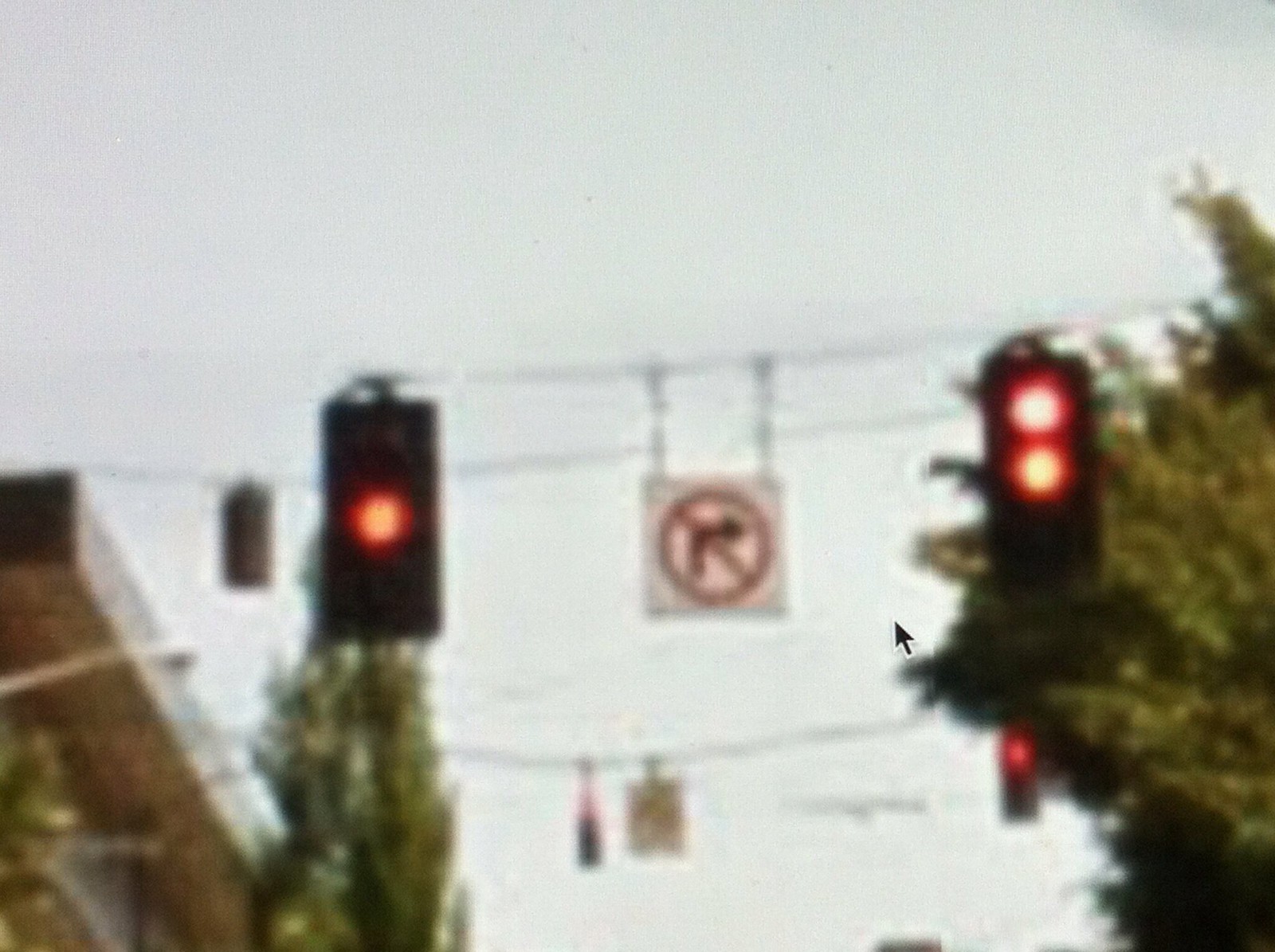This outdoor, daytime photograph, taken in bright but overcast conditions, depicts a slightly grainy and blurry urban scene dominated by rectangular traffic lights and trees. Two horizontal cables stretch from left to right across the center of the image, supporting two distinctly rectangular traffic lights. The left light features a circular red light in the center, appearing more orange-red due to the image's blur. To its right, a second traffic light displays a circular red light at the top and an orange light at the bottom. Both lights are filled and edged in black.

Between these traffic lights, also suspended from the cables, is a square sign, marked with a red circle and a diagonal line through it, overlaying a black arrow pointing to the right, indicating no right turn. In the backdrop, additional traffic signals can be seen hanging from another wire, displaying red lights.

On the lower left side of the image, there’s a partial view of a roof belonging to a gray and light brown building, accompanied by small evergreen trees stretching upward. Towards the center-left and extending behind the traffic lights, a larger evergreen tree stands prominently against the bluish-gray sky. Another full-grown evergreen tree is also situated on the right edge of the photograph. The overall scene represents a typical urban street setting, captured in a soft, slightly out-of-focus manner.